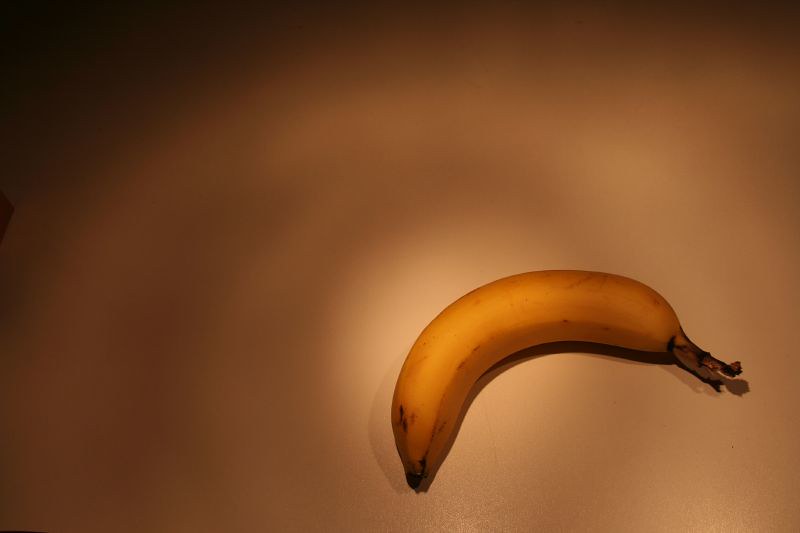This image features a single yellow banana set against a dynamic gradient background. The gradient transitions diagonally, starting from a deep black in the top left corner and gradually lightening to a soft tan in the bottom right corner. The banana, positioned slightly off-center, leans towards the bottom right corner, with its stem pointing downwards. Gentle curvature characterizes the banana, adding a naturalistic touch. Subtle brown markings are visible at its base, further emphasizing its realism. The overall composition, enhanced by the gradient and the strategic lighting, creates a spotlight effect that draws the viewer's attention directly to the banana.